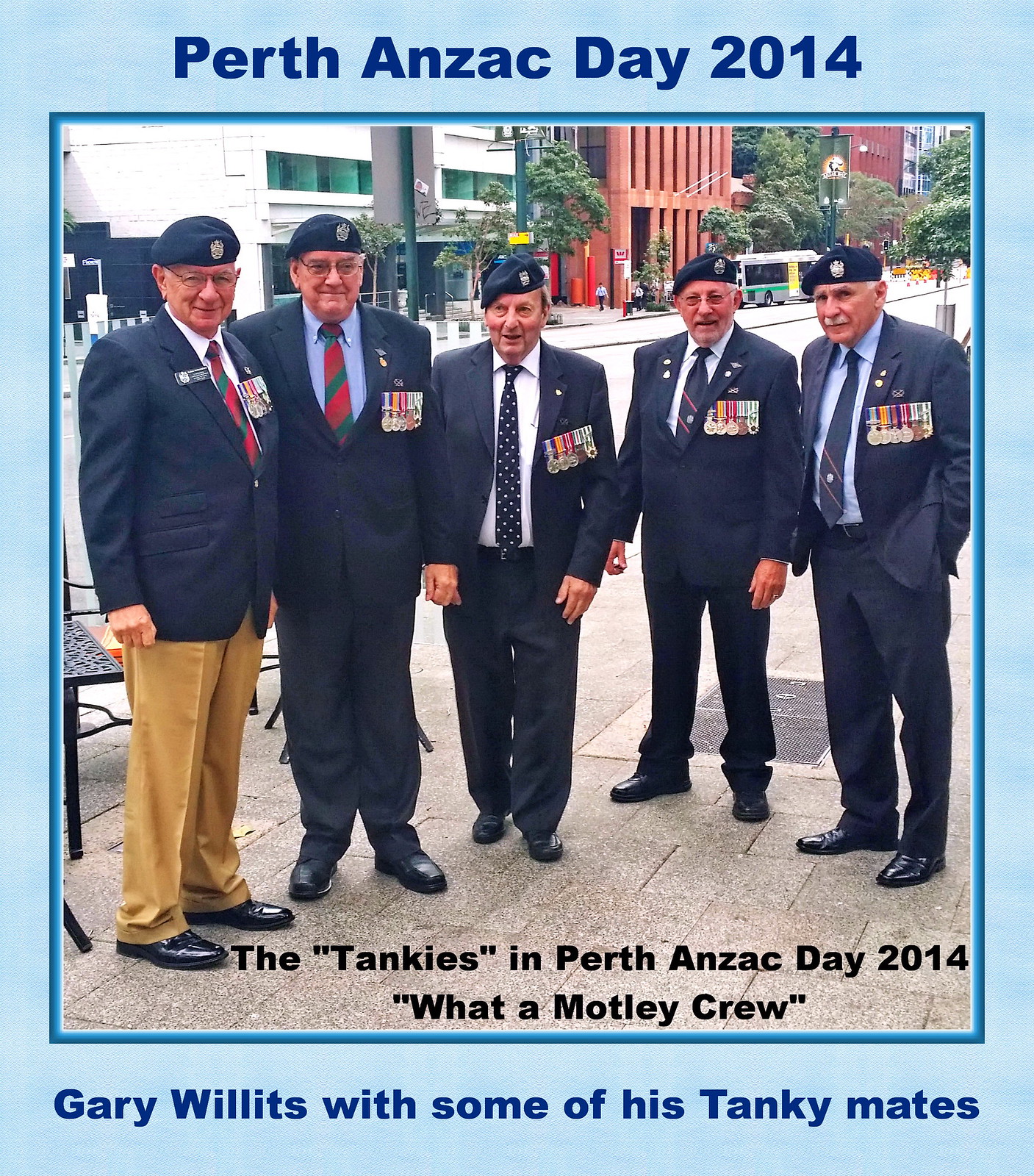The image features five elderly veterans, proudly wearing an array of military medals on the right side of their blue suit jackets, along with beret hats. They stand together on a concrete brick sidewalk, facing the camera. The men are dressed in various colors of pants, with most in blue or black and one in khaki. The photo is framed with a light blue border, with "Perth Anzac Day 2014" written at the top and "Gary Willits with some of his tankie mates" at the bottom. Superimposed text within the image reads, "The Tankies in Perth Anzac Day 2014. What a motley crew." In the background, a street and several multi-story buildings can be seen, suggesting an urban setting in downtown Perth. The veterans, well-past their prime years, stand as a testament to their service and camaraderie on this commemorative day.